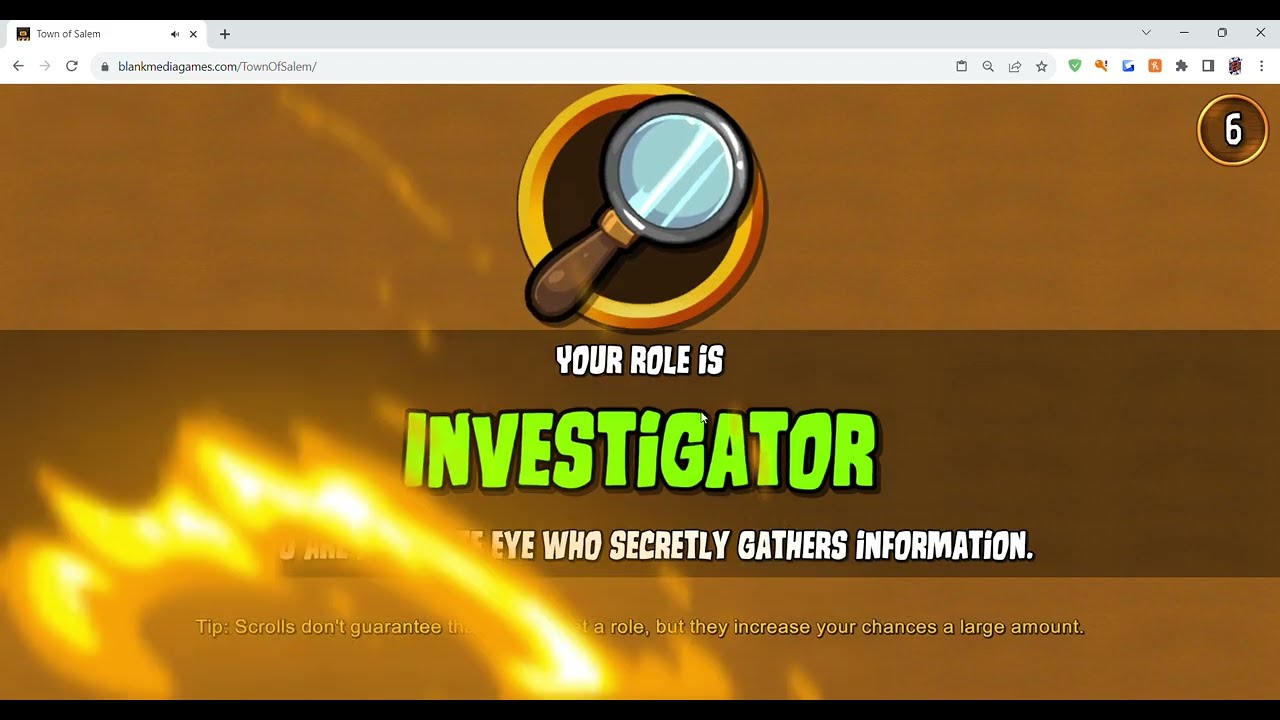In this screenshot of a browser window displaying the game "Town of Salem" hosted on blankmediagames.com, the URL is partly visible. The entire browser interface, including little icons and clickable elements unrelated to the site, frames the image. Central to the webpage is a prominent magnifying glass inside a gold circle, symbolizing the investigator role in the game. Text on a small banner below the magnifying glass declares, "Your role is investigator." Some of the accompanying explanatory text is partially obscured by animated flames, revealing phrases like "I who secretly gathers information." Another line reads, "Tip: scrolls don't guarantee that a role but they increase your chances a large amount." The background is divided into distinct horizontal sections with a tan bar occupying a third of the screen, a very dark brown bar, another tan bar, and a solid black bar. The color scheme primarily includes white, gray, yellow, orange, green, and black, all contributing to the themed aesthetic of this game's user interface.